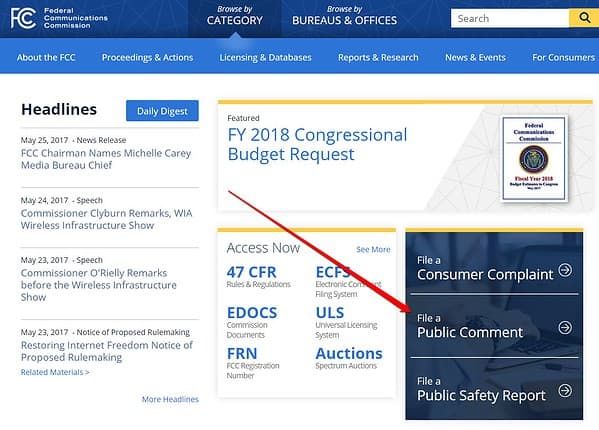Screenshot of the Federal Communications Commission (FCC) Website Interface

This detailed screenshot captures the user interface of the Federal Communications Commission (FCC) website as viewed on a computer. 

At the top of the page is a banner displaying the FCC logo on the left, with the text “Federal Communications Commission” prominently featured. Although the web address is not visible, familiar navigation elements confirm it is an official website.

Directly below the banner is a series of navigation tabs allowing users to browse by category. Following this is a section labeled “Headlines and Daily Digest,” showcasing various headlines from May 2017. To the right of this section, a notable header reads “FY 2018 Congressional Budget Request.”

A prominent red arrow pointing downward directs attention to a link labeled “File a Public Comment.” Additional sections below this offer options for users to file a Consumer Complaint, a Public Comment, or a Public Safety Report.

In the upper right-hand corner, a search box is available for quick navigation, alongside a link labeled “Browse by Bureaus and Offices," encouraging users to explore different areas of the FCC.

This comprehensive interface layout ensures users can easily navigate through the information and services provided by the FCC.